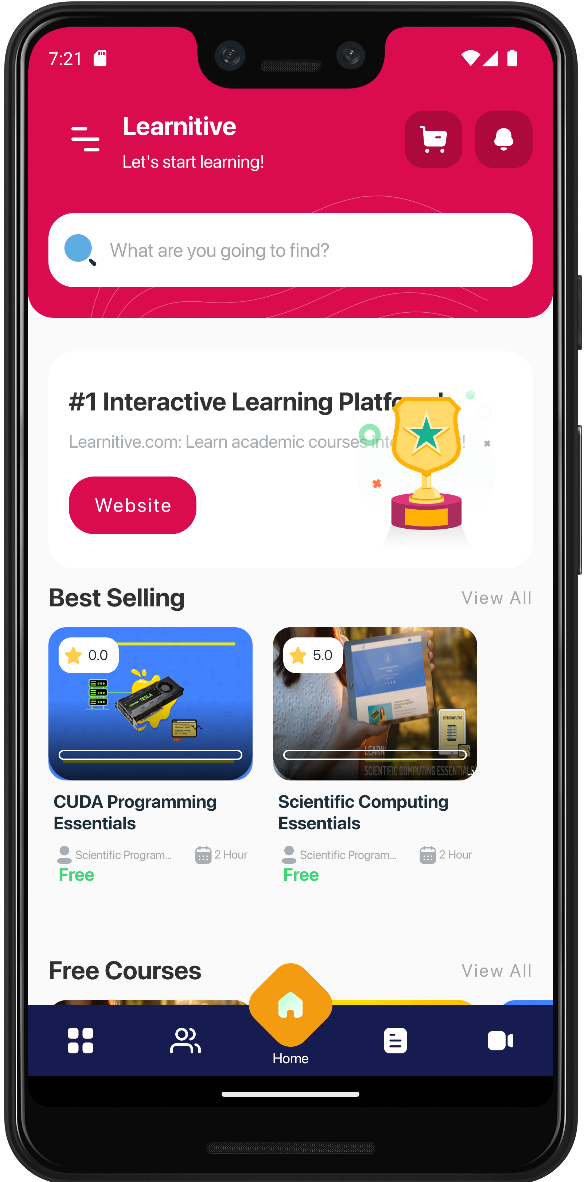The image depicts a cell phone screen showcasing an educational platform interface. The top section of the phone's display is red, containing standard icons such as cell and Wi-Fi signal bars, a full battery indicator, and the time, 7:21 AM. 

Immediately below these icons is the platform's name, "Learnative" (L-E-A-R-N-I-T-I-V-E), followed by the slogan "Let's start learning." Adjacent to the platform name are icons for a shopping cart and notification bell. 

A prominent white search bar, labeled "What are you going to find?" and featuring a magnifying glass icon, is displayed on a white background. Below this search bar, the text reads "Number One Interactive Learning Platform. Learnative.com. Learn Academy Courses." Next to this text is a graphic of a trophy on a pedestal with a green star, indicating an award or achievement. 

Further down, there's a red button labeled "Website" in white text. The next section promotes specific courses: 
- "Best-selling CUDA Programming Essentials: Scientific Computing Programming - 2 hours free." 
- "Scientific Computing Essentials: Scientific Programming - 2 hours free."

A "View All" button is visible below these course descriptions, followed by the text "Free Courses," though the details are partially cut off. 

The bottom portion of the screen features a navigation bar with icons for four sections: two people, a home icon (in orange), a page, and a video camera. The screen is topped off with a white line indicating the bottom of the phone's interface.